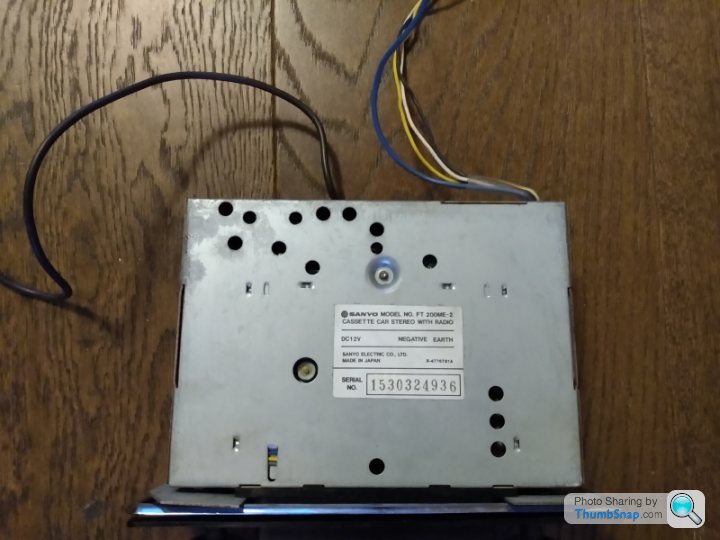This is an amateur photograph taken indoors, featuring a detached car stereo unit, specifically a Sanyo model FT200ME-2 Cassette Car Stereo with Radio, displayed upside down on a richly stained, dark brown hardwood floor. The image is a square, full-color shot taken from above, with the lighting appearing dim. The metallic gray device has several black ventilation holes visible and is labeled with a white plaque in the center bearing the black text: "Cassette Car Stereo with Radio, DC-12V, Negative Earth," and the serial number "1530324936." Multiple colored wires, including black, blue, yellow, and white, are seen protruding from the bottom of the device. In the bottom right corner of the image is a small logo for Thumbsnap.com, featuring a cartoon magnifying glass in black, white, gray, and blue.